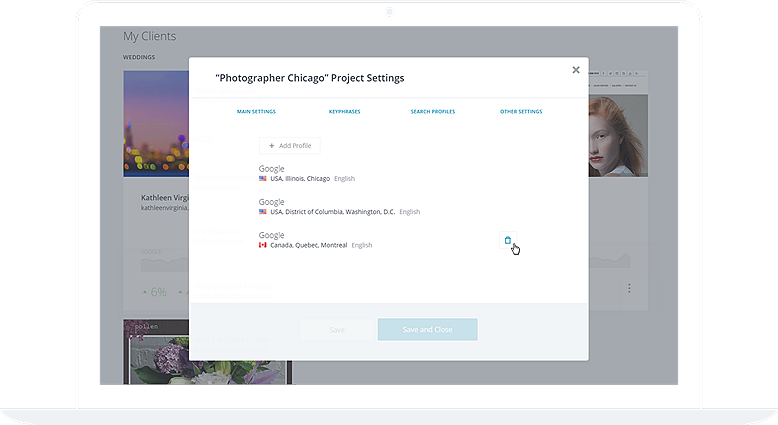The image is a screenshot of a website showcasing a photographer's portfolio. The background features a gray page with the title "My Clients" and a section heading "Weddings," alongside various photos, though only one is clearly visible. On the side of the webpage, there's a photograph of a woman with red hair, presumably the photographer.

In the upper part of the webpage, a pop-up partially obscures the main content. This pop-up is titled "Photographer Chicago Project Settings" and includes an 'X' button for closing. The pop-up contains four clickable tabs: Main Settings, Key Phrases, Search Profiles, and Other Settings. 

Beneath these tabs, there is a small box with a plus sign labeled "Add Profile." Below this, there's a list of three profiles:
1. Google, American Flag, USA, Illinois, Chicago, English.
2. Google, American Flag, USA, District of Columbia, Washington, D.C., English.
3. Google, Canadian Flag, Canada, Quebec, Montreal, English.

The cursor is pointed at a trash can icon next to the third profile. At the bottom of the pop-up, there are two buttons—Save and Save and Close—which are both grayed out. Additionally, a background photo of flowers is faintly visible at the bottom of the webpage.